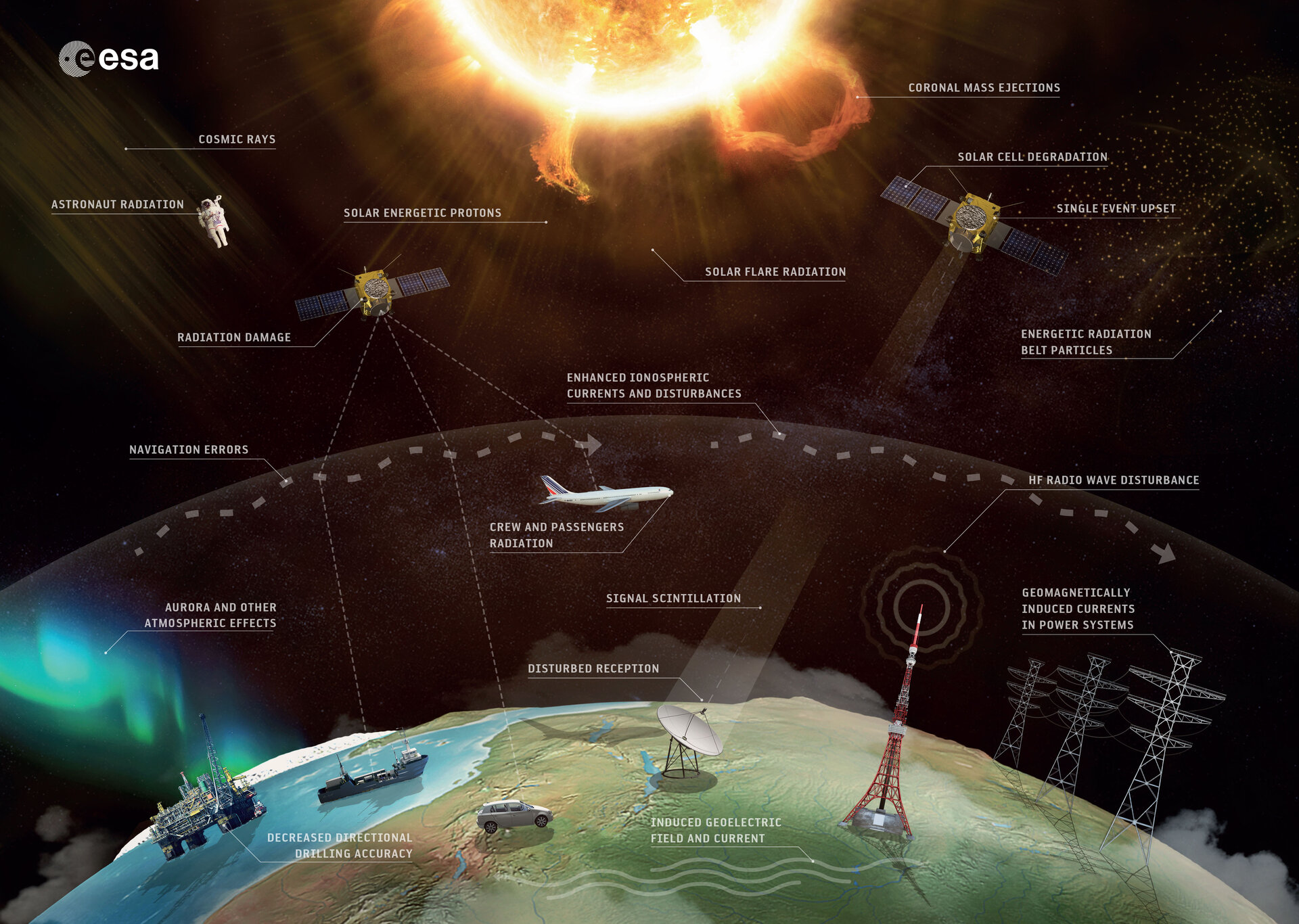The detailed diagram illustrates the Earth’s atmosphere and its interaction with space phenomena. In the lower section, the Earth's curved surface is depicted with various key elements such as an oil rig in the ocean (bottom left), a ship, a car, a large communication tower emitting radio waves, and large electrical power lines (bottom right). Additionally, a vehicle and a commercial plane are visible navigating above the Earth's surface. The translucent sphere around the Earth signifies the atmospheric layer, dotted with navigation error indicators.

In the upper section, the vast black space is highlighted by the enormous, fiery Sun occupying the top center, emitting vivid beams and flares. Detailed labels indicate the Sun-related phenomena: "solar energetic protons," "solar flare radiation," and "coronal mass ejections," with arrows pointing towards the emanating beams and flames.

Notably, the diagram includes two satellites, each labeled for "solar cell degradation" and "radiation damage," floating beside the Earth. An astronaut appears at the top left, annotated with "astronaut radiation." The presence of cosmic rays and energetic radiation belt particles are also noted.

Additional atmospheric interferences are marked around the diagram, including "geomagnetically induced currents in power systems," "enhanced ionospheric current disturbances," "HF radio wave disturbance," "disturbed reception" near a satellite dish, and "decreased directional drilling accuracy" adjacent to the oil rig. Furthermore, "aurora and other atmospheric effects" and "crew and passenger radiation" impacts on the commercial plane are specified.

Overall, the complex interaction between the Sun's emissions and Earth's technological and atmospheric systems is meticulously detailed with comprehensive labels and arrows. The presence of "ESA" in the top-left corner signifies the European Space Agency's endorsement or origin of the illustration.